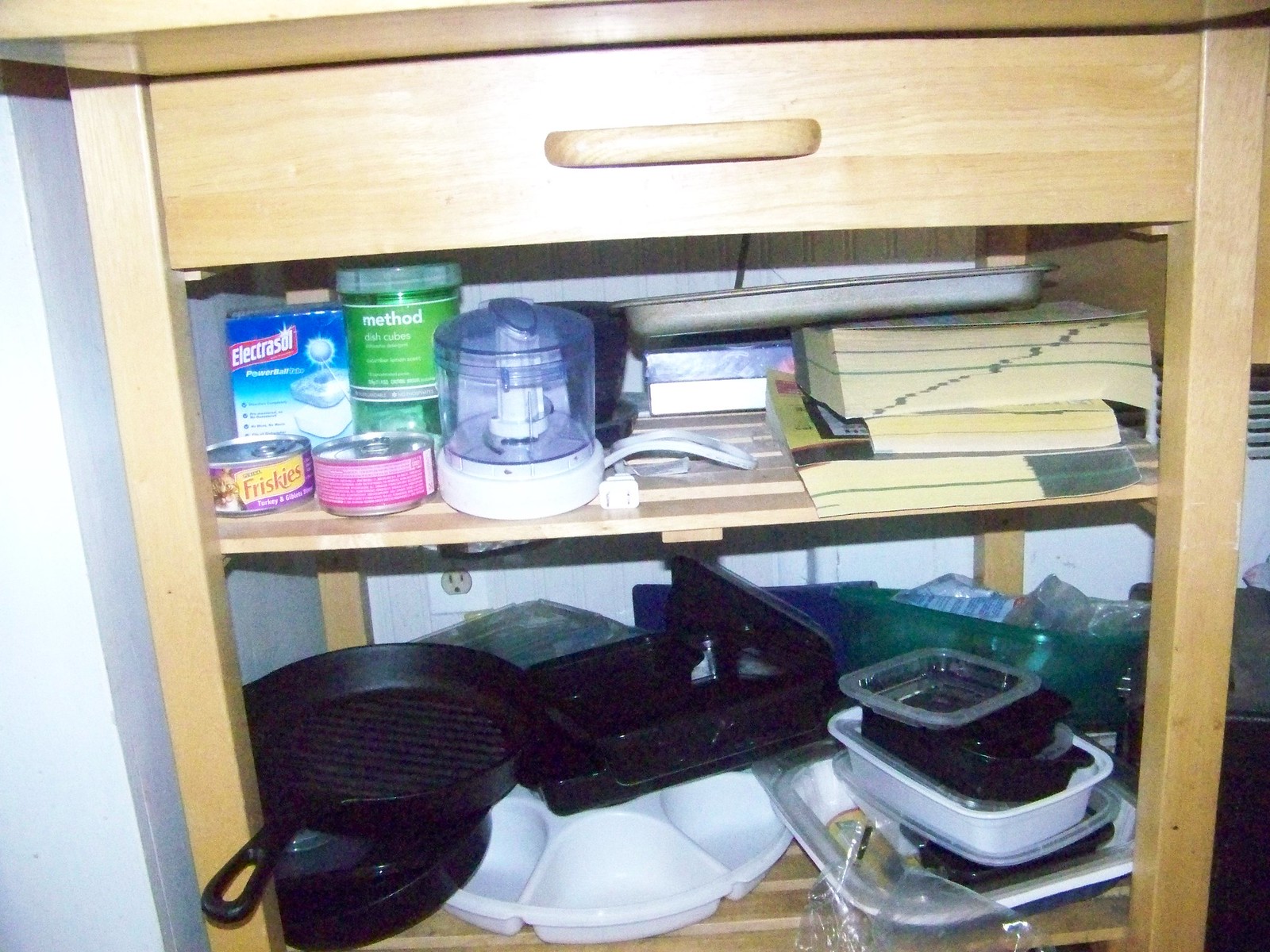The photograph depicts a wooden kitchen shelf unit, left unpainted to reveal its natural wood grain. This multifunctional shelf features a closed drawer with a wooden handle at the top. Below the drawer, a shelf holds several cans of cat food, a small appliance possibly used for food processing, and household cleaning products such as Electrasol and Method dish cubes.

Further down, there’s a metal sheet pan, alongside two stacked phone books. The lower section of the unit contains an assortment of kitchen items including various pots and pans, with a notable cast iron pan. Additionally, there's a white multi-compartmentalized tray suitable for serving different types of food like fruits or dips. A green container with unidentified contents occupies a corner of the shelf. The overall cluttered yet organized setup suggests this piece of furniture is indeed utilized in a kitchen environment.